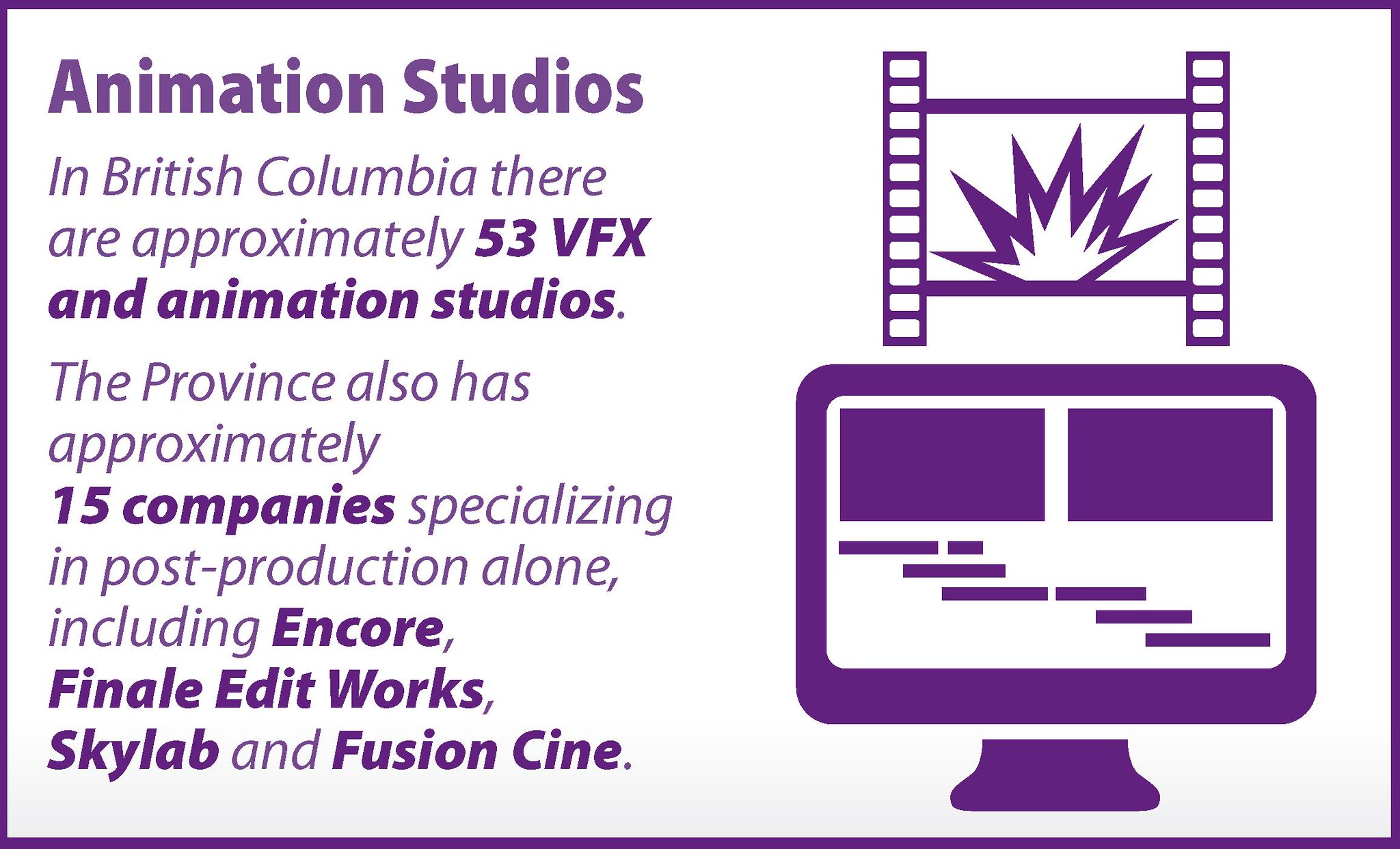The infographic features a clean white background with a distinctive purple border. On the left, purple text prominently reads "Animation Studios," with further detailed information below. It states, "In British Columbia, there are approximately 53 VFX and Animation Studios," highlighted in bold purple. Subsequently, it mentions, "The province also has approximately 15 companies specializing in post-production alone, including Encore, Finale, Editworks, Skylab, and Fusion Cine," with the 15 companies and their names similarly emphasized in bold purple text.

Moving to the right side of the infographic, there are two distinct graphic elements. The upper graphic depicts a film reel silhouette, detailed with white squares on the left and right sides and two horizontal lines, one above and one below. Centrally featured within this graphic is a stylized explosion silhouette in purple and white, representing a frame from a film reel. Below this is the second graphic: a computer monitor silhouette in purple, with a white screen. Purple squares adorn the top left and right of this design, complemented by horizontal lines below, and the computer base is also illustrated in purple. The entire design creates a cohesive, visually appealing representation of British Columbia's animation and post-production industry.